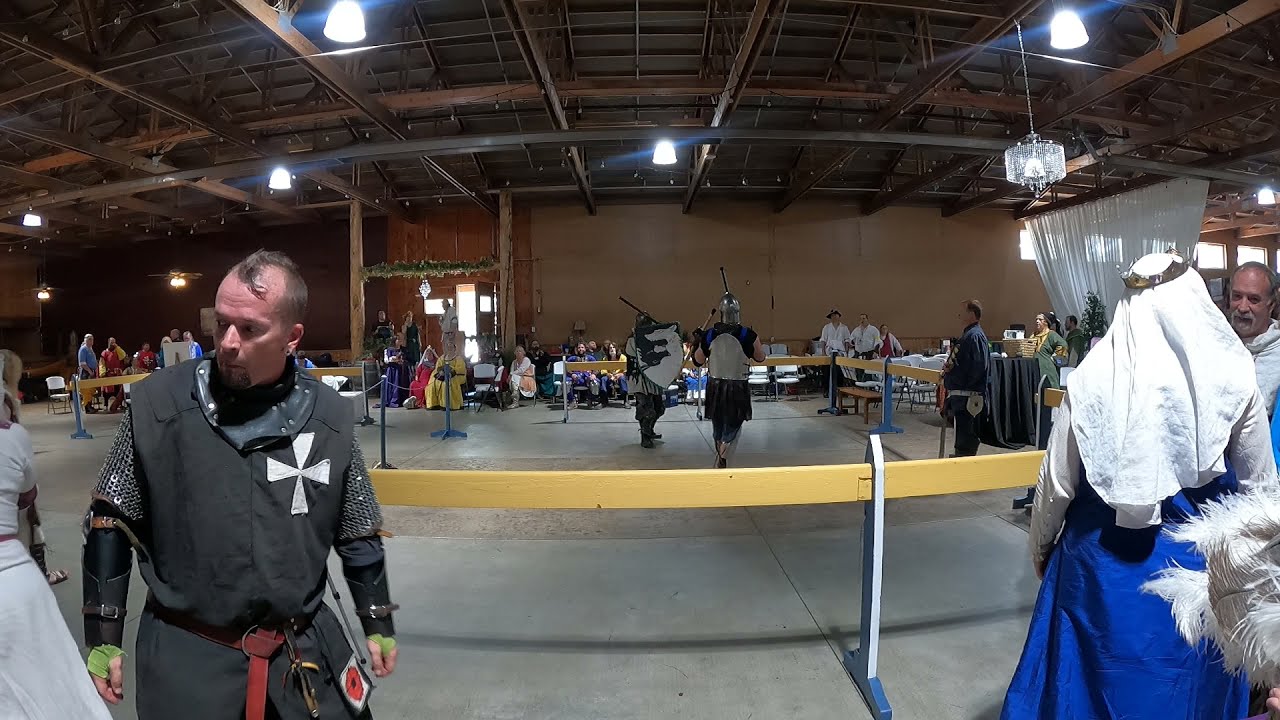In this detailed indoor scene set within a warehouse-style building, a medieval-themed event unfolds, likely a renaissance festival or similar gathering. The focal point is a Caucasian man standing prominently in the foreground. He wears a black tunic adorned with a white cross and chainmail sleeves, complemented by black leather gauntlets and a red leather belt tied in front. His hairstyle is a somewhat balding, sloppy mohawk, and he sports a goatee and mustache. To his right, a woman, possibly resembling Maid Marian, is seen from behind, donned in a blue dress and a white shawl, topped with a white headdress.

The background reveals a bustling fairground on a concrete floor. The arena-like area is fenced off and features participants in medieval attire, engaging in mock battles with wooden sticks instead of swords. Some people are dressed as knights, while others appear to be spectators in colorful robes, suggesting a rich tapestry of role-playing and reenactment. The atmosphere is enlivened by details like hanging vines on the supports near the main entryway. Far in the distance, figures potentially representing a king and queen, and a monk can be discerned. The wide-angle lens captures the immersive depth of the scene, curving some elements like white feathers in the foreground while providing a detailed view of the festivity.